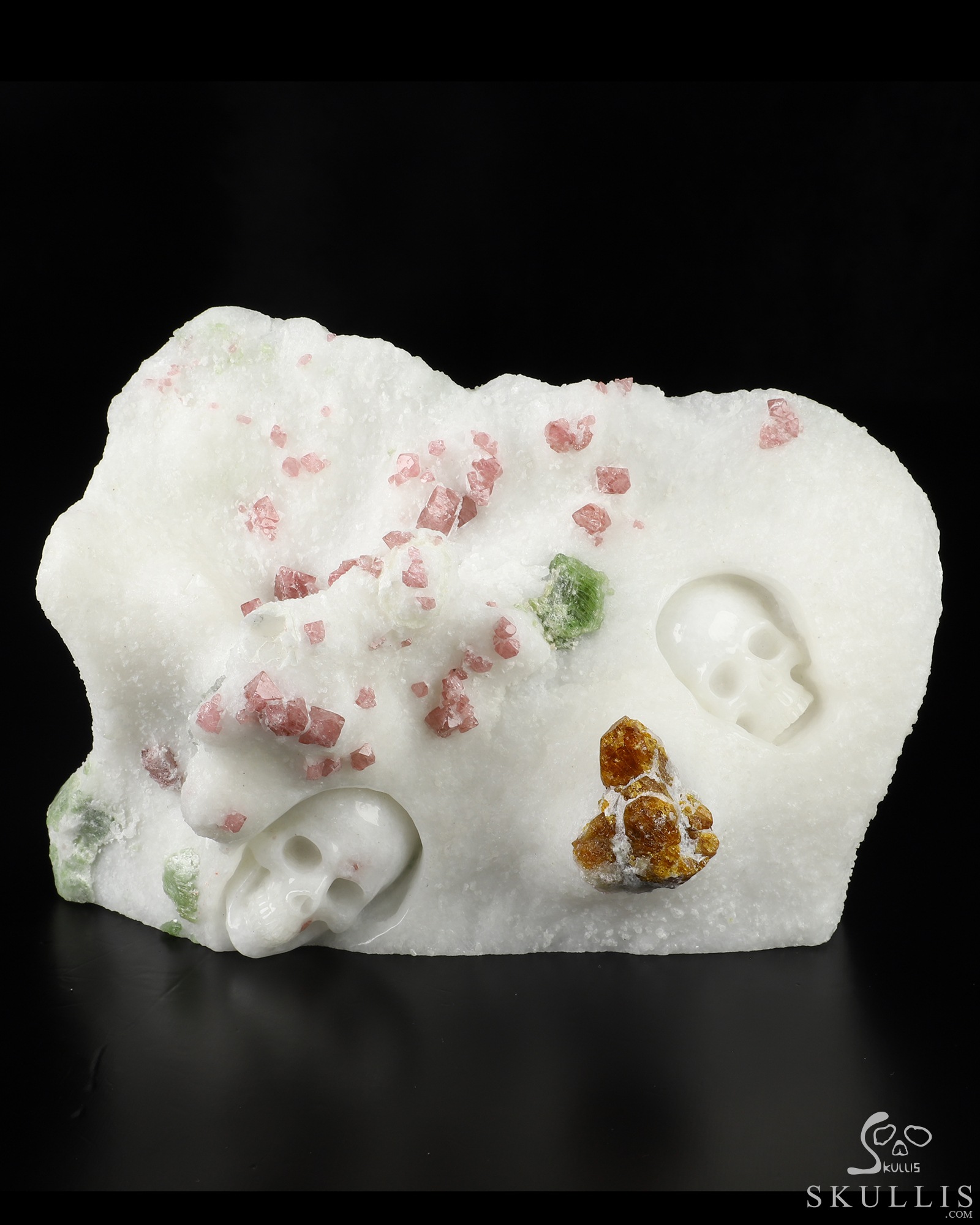The image depicts a white, crystal-like figurine with a complex texture that resembles compressed sugar or powder. Embedded within the figure are two prominent white skulls and scattered about are small decorative pieces in various colors, including pink, red, yellow, and green. These decorations might be small rocks, crystals, or candy pieces. Additionally, there is a cluster of brown rock and another green element located around the middle-left area. The figurine is set against a stark black background, enhancing its striking appearance. In the lower right corner, the logo "Skullis" (spelled S-K-U-L-L-I-S) appears, featuring a skull-like design, framing the piece as potentially a decorative or themed item, possibly for Halloween.